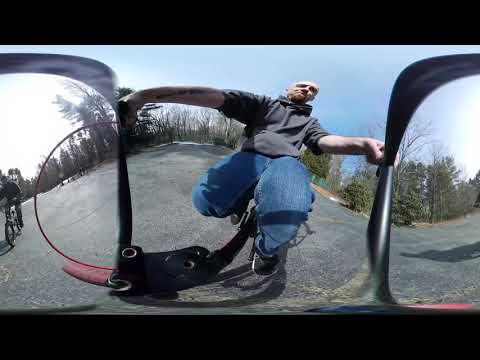The image depicts a balding man with a stubble or goatee, wearing a gray or dark hoodie with rolled-up sleeves, blue jeans, and black sneakers, riding a bike. The photo, taken from a slightly low perspective with the camera positioned between the handlebars, gives a slightly distorted view focusing on the man. He seems to be holding on to the bike's handlebars while pedaling on a paved road lined with trees under a light blue sky scattered with clouds. A green fence is visible behind him, lining the tree border, and another biker is approaching from the opposite direction. The season appears to be late in the year, as some trees have lost their leaves, indicating a likely autumn setting.